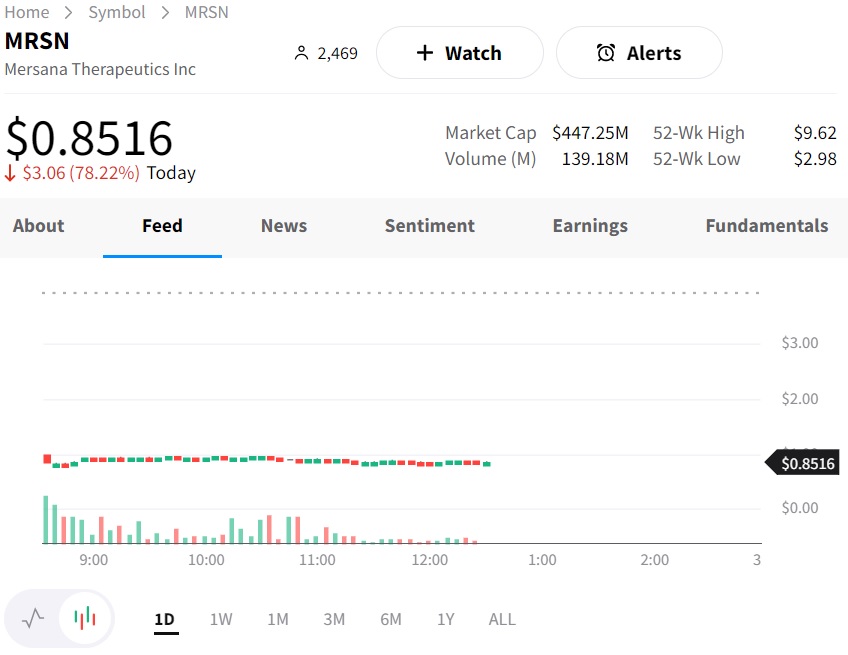**Screenshot Overview of MRSN Stock Performance**

This detailed screenshot captures a stock performance chart of Marsana Therapeutics, Inc. (Ticker: MRSN) over a single day. The interface includes multiple elements to convey crucial information:
 
- **Breadcrumb Navigation**: Located at the top left corner, it shows a "Home" symbol followed by 'MRSN,' which stands for Marsana Therapeutics, Inc.
  
- **User Icon**: To the right of the company name, a silhouette icon is displayed with the number 2469 next to it, indicating the number of users monitoring this stock. Nearby are two buttons: one for adding the stock to a watchlist and another for setting alerts.
  
- **Stock Chart**: The main chart depicts MRSN's stock performance from 9:00 AM to 3:00 PM. The vertical axis ranges from $0 to $3, and the stock is currently priced at $0.85, reflecting a significant decline of 78.22% for the day.
  
- **Key Metrics**: On the far right side, two columns of essential statistics are provided:
  - Market Cap: $447.25 million
  - 52-Week High: $9.62
  - Volume: 139.18 million
  - 52-Week Low: $2.98

- **Tab Navigation**: Below these statistics is a row of tabs, offering various information categories including Feed, News, Sentiment, Earnings, and Fundamentals. The 'Feed' tab is currently selected and highlighted in blue.